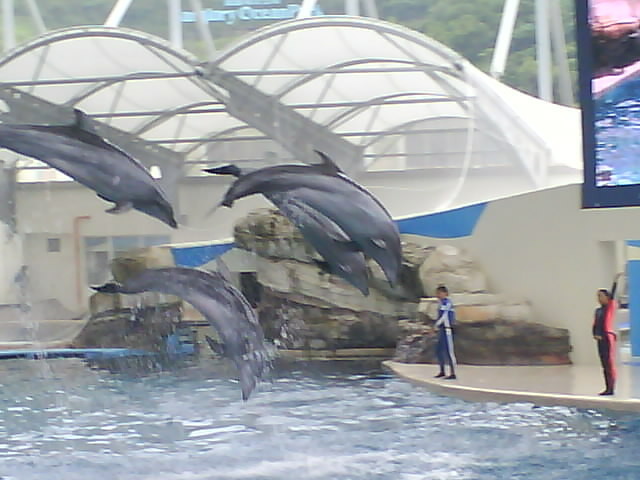In this action shot from a marine-themed amusement park, reminiscent of SeaWorld, we observe an energetic dolphin performance. The image captures four dolphins, characterized by their light grey hue, mid-leap, their bodies arched gracefully with tails up and noses pointed toward the water. They are performing in a pool, with a stage behind them where two trainers—one in a blue wetsuit with white accents and the other in a black wetsuit with a red stripe—are poised. The background features a sizeable digital screen in the upper right-hand corner, a white canopy providing shade above the dolphin habitat, and decorative rock structures to the right. A sign in the backdrop hints at "Ocean Park," completing this lively scene.